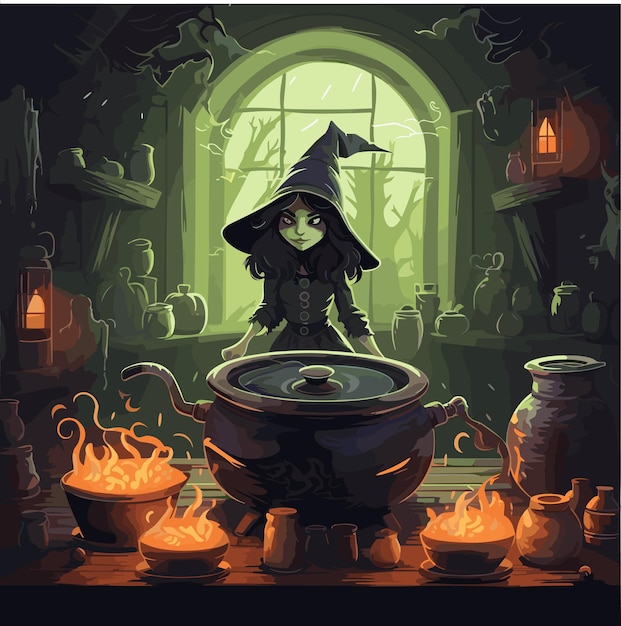This digital drawing captures a whimsical, yet detailed, cartoon-like depiction of a young witch in her Halloween-themed kitchen. The witch is adorned in traditional attire, featuring a tall, pointy black hat that is wider than her shoulders, a black dress with mid-forearm sleeves, and huge buttons down the front. Her shoulder-length hair is brown, contrasting with her very pale, almost white face. She stands in front of a large, black cauldron positioned on a wooden table; the cauldron’s lid is on, hinting at mysterious contents inside.

Around the cauldron, there are three bowls with flaming yellow and orange fires, contributing to the room's eerie ambiance. The kitchen is cluttered with various sized bowls, containers, and potion jars, some open and some closed, strewn about the shelves along the walls. Lanterns with candles emit a warm, yellow glow, adding to the spooky atmosphere. Behind the witch, an arched window casts a light green hue into the room, intensifying the eerie mood. Through the window, the silhouettes of dead trees are visible, enhancing the overall Halloween theme. The carefully detailed elements, from the fiery bowls to the potion-filled shelves, create a richly immersive scene.